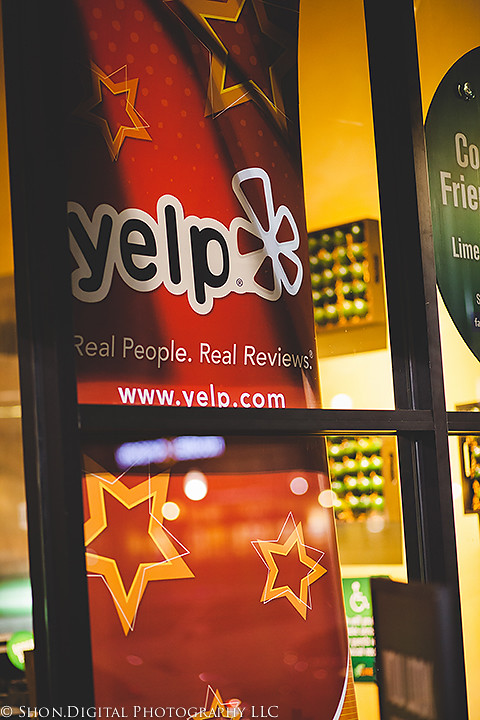In this image, we are looking through a black paned glass window into a room filled with various elements and decorations. The main focus is a large, vertically hung red poster positioned in the center. The poster features gold and yellow star outlines with white thin line star accents on top, blending into the same red hue as the background. At the top of the poster, there are faint light red dots adding texture to the backdrop. Dominating the center is the black Yelp logo, accompanied by an asterisk-like symbol formed by red pie slices, all outlined in white. Beneath the logo, in white text, it reads "Real People, Real Reviews," followed by the website URL, "www.yelp.com." In the lower left-hand corner of the poster, in small print, it says "Copyright Sean, digitalfotography LLC." On the right window pane, there is part of another circular green poster with cut-off text that reads "CO" and "FRIE." Additional visual elements inside the room, including a yellow backdrop and a cabinet on the wall, contribute to the rich details of the scene. The photograph appears to be taken from outside, capturing a moment through the window.